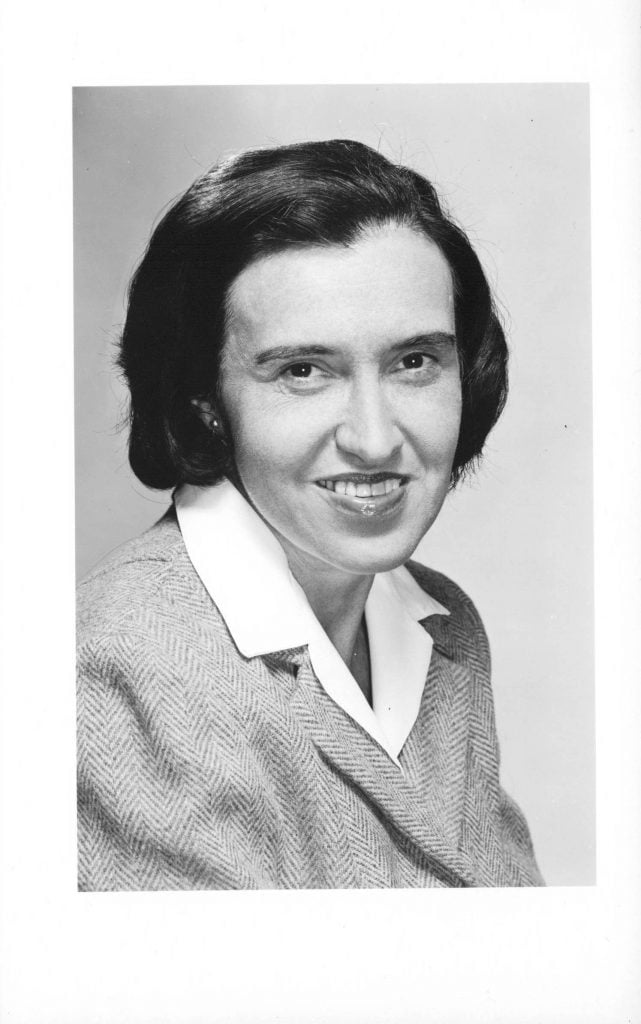This black and white portrait, evoking the style of the 1930s or 1940s, features a middle-aged woman looking directly at the camera with a warm smile that exposes her upper teeth. Her short, dark hair is neatly parted on the left side and covers her ears, adding to the period feel of the image. She dons a white collared blouse underneath a light-colored tweed or sports jacket, the meticulous arrangement of her attire indicating the portrait's professional nature. The background is plain and subtly illuminated, enhancing the focus on her symmetrical face with minimal makeup and no visible jewelry except for a possible round earring in her right ear. Her head is slightly tilted to the right, contributing to the nuanced expression captured in this carefully composed photograph.